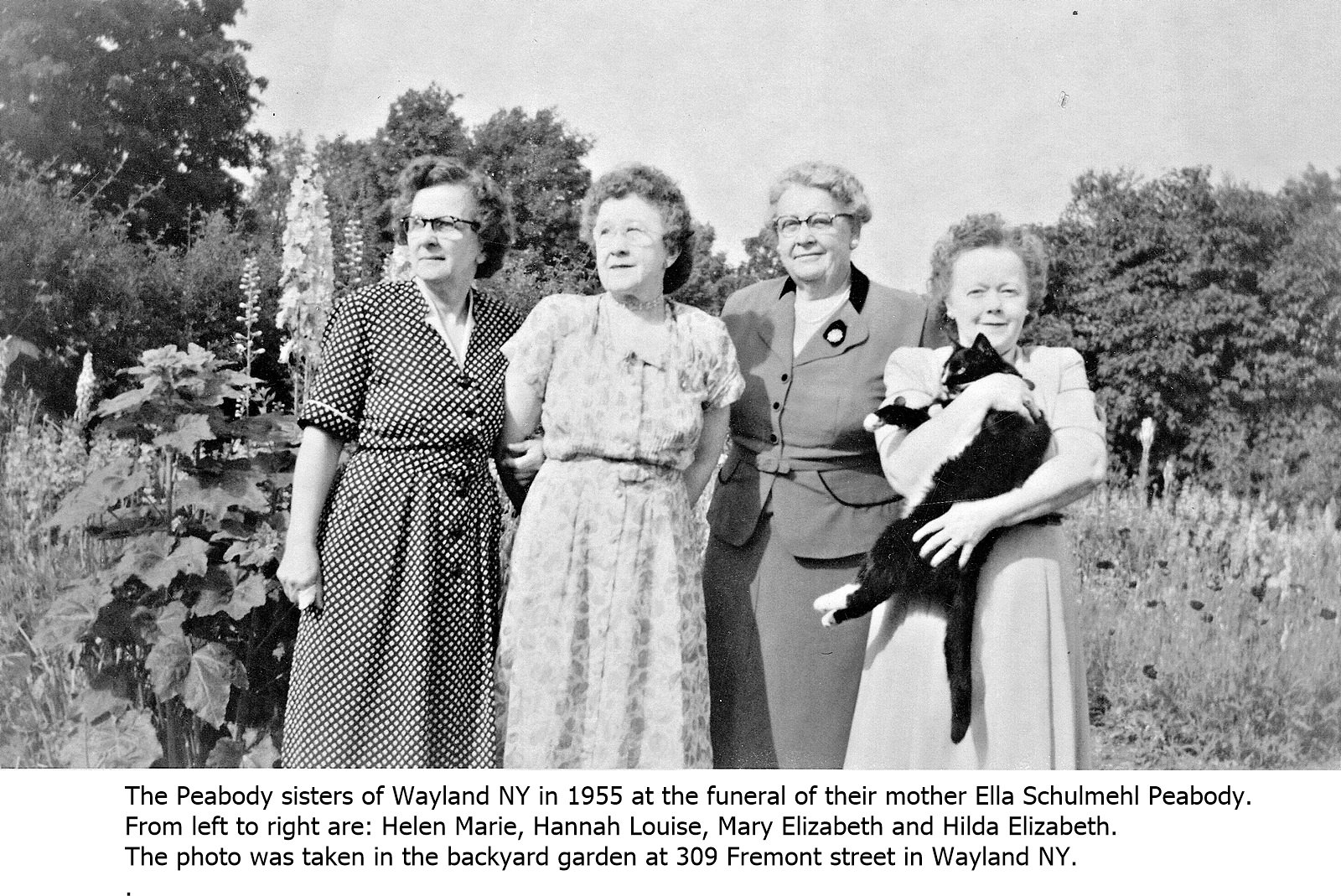This is a detailed black and white photograph taken from an article or a magazine in a book. It features four older women standing outdoors in the backyard garden at 309 Fremont Street, Wayland, New York, on a clear, sunny day in 1955. They are identified as the Peabody sisters—Helen Marie, Hannah Louise, Mary Elizabeth, and Hilda Elizabeth—at the funeral of their mother, Ella Schumel Peabody. 

The four women are standing in front of a field with large, fully-leaved trees in the background and a noticeable play of shadows indicating the sunlight. From left to right, Helen Marie is wearing a white polka dot dress and glasses; Hannah Louise is in a light floral design dress and glasses; Mary Elizabeth is dressed in a dark grayish business suit with glasses; and Hilda Elizabeth is in a white dress holding a black cat with white paws, and is the only one not wearing glasses.